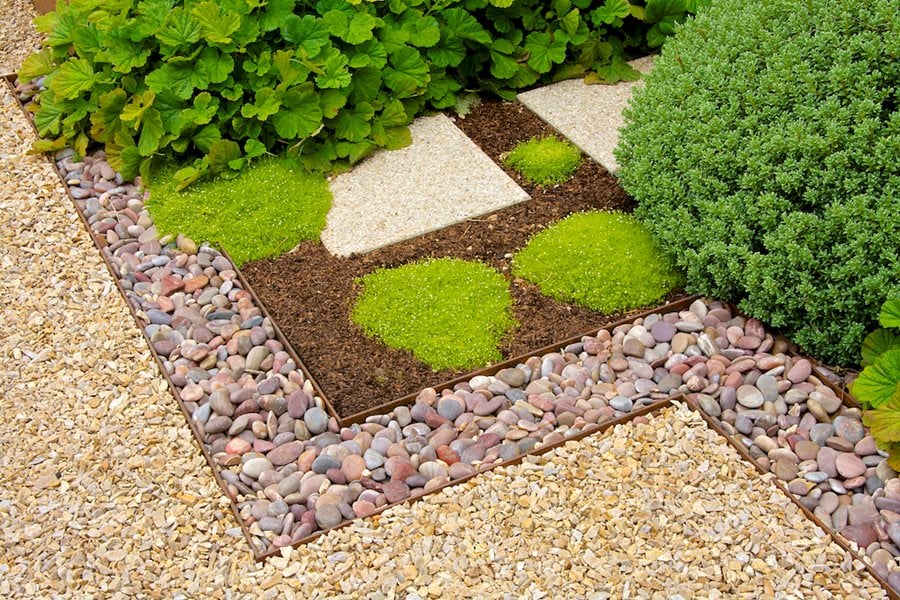The image captures a meticulously landscaped garden that blends a rock garden with lush greenery. In the forefront, a section of light yellow to white pebbles, evoking a beachy feel, is bordered by larger, multicolored stones ranging from browns and grays to whites. Another distinct border separates these pebbles from an area of dirt adorned with small patches of grass and strategically placed stepping stones. 

Several types of green bushes populate the garden, including three with large leaves and a smaller shrub. To the right, a lush green bush dominates the top right corner, alongside more greenery cascading from the top edge about a quarter way down. A diagonal pathway, lined with round pebbles forming distinct right angles, traverses the garden. 

In the middle of this well-designed space, a square stone is set in mulch that intermingles with small, wiry green plants, contributing to the garden's serene ambiance. The mulch, resembling wood chips, adds texture to the landscape. Overall, the garden showcases a harmonious blend of natural elements and careful design, creating a visually appealing outdoor sanctuary.